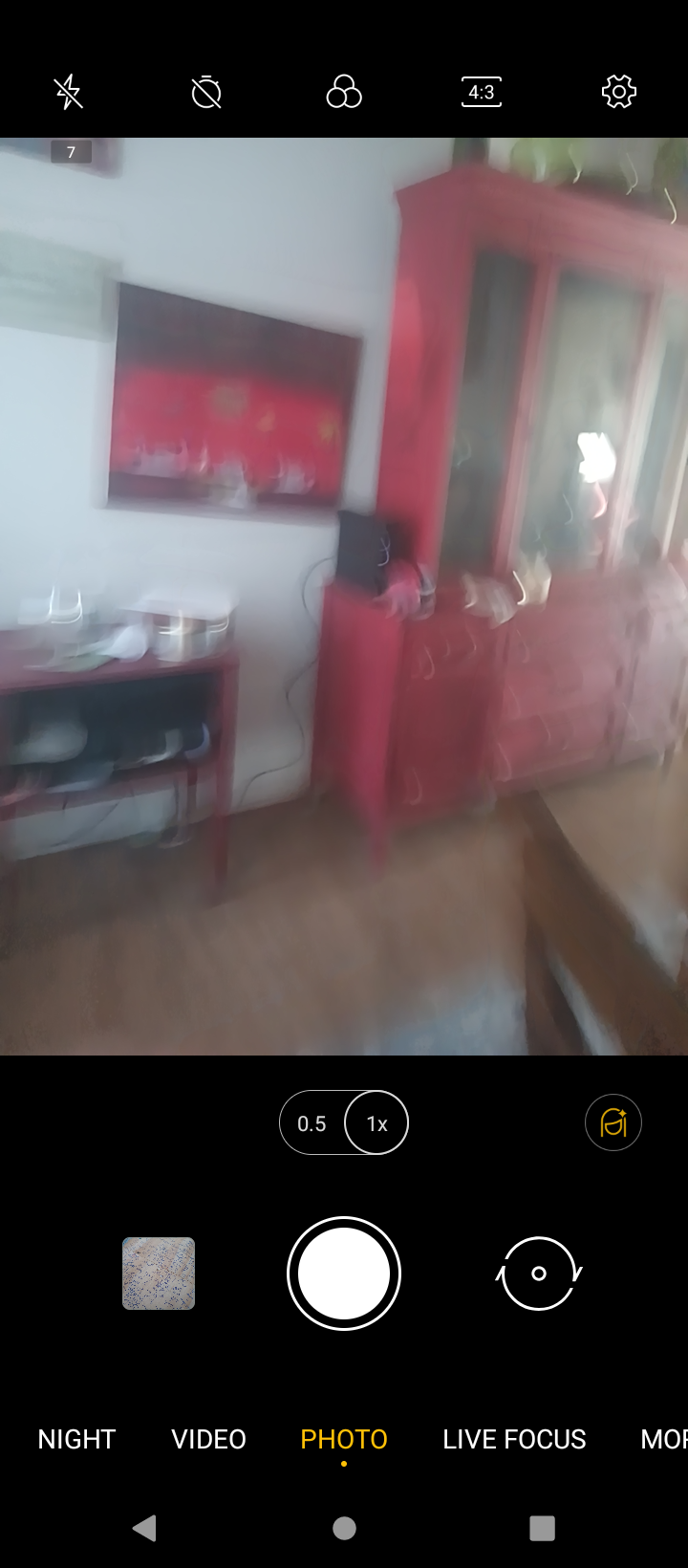In the blurry image captured on an iPhone using a photo editing or camera app, the interface displays options at the bottom including "night," "video," "photo," and "live focus." A white record symbol, consisting of a solid circle with a white outline, is prominently featured, accompanied by arrows encircling it on the right side and a square icon on the bottom left. The scene within the photo is indoors, showcasing a room with a white wall adorned with a crooked red picture on the left. The wooden floor is visible, with a small red table on the left side of the image. Dominating the center is a large red cabinet with a glass front, possibly with items placed on top. A seat is positioned at the bottom right, contributing to the overall composition of the room.